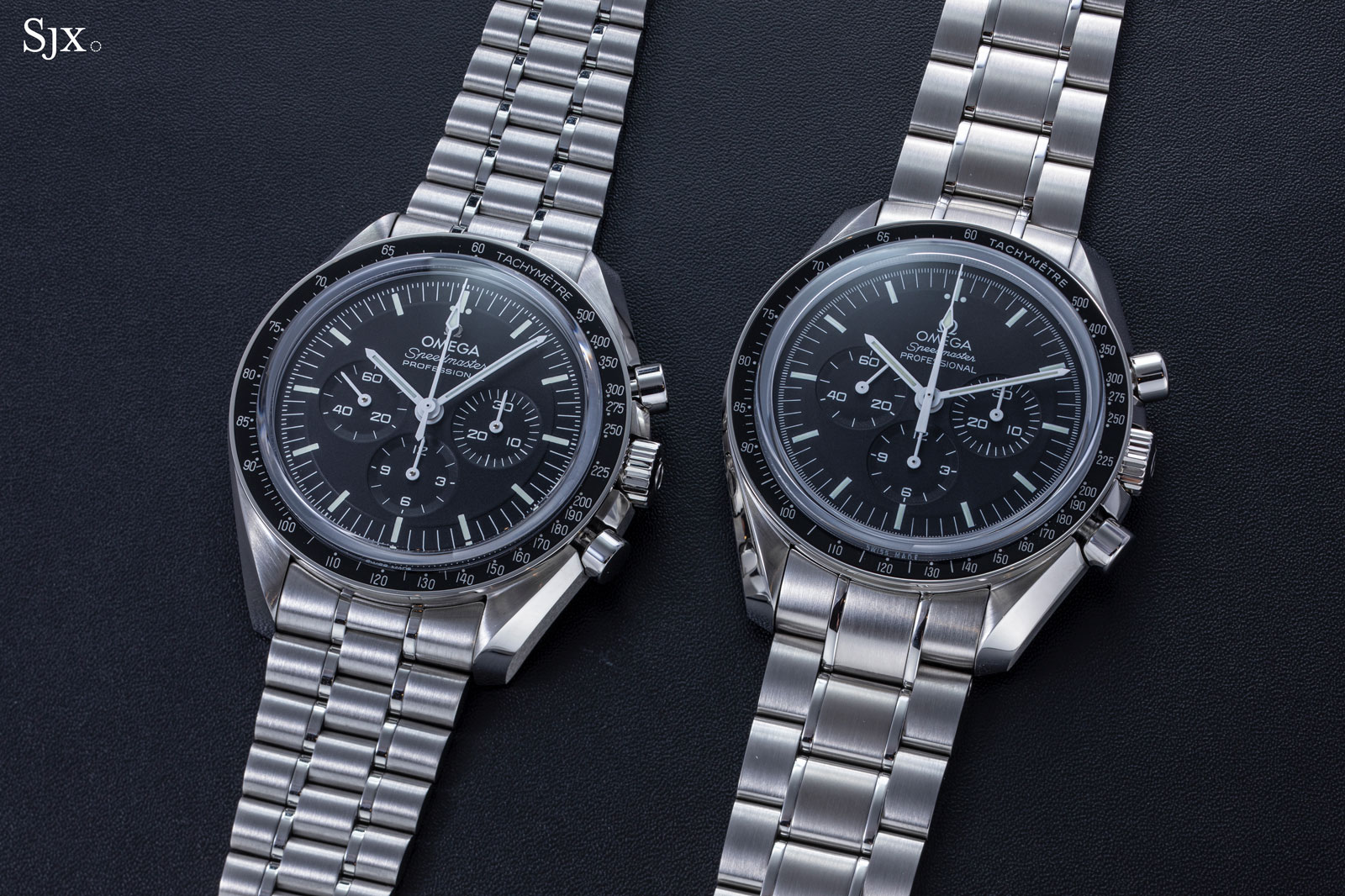The image displays two Omega wristwatches laying on a plain black surface, under the white letters "SJX" followed by an unfilled circle. Both watches share a similar design, featuring main clock faces along with three smaller subdials, although their specific functions are not labeled. The bands of both watches are silver with a pattern of interspaced coils. The watch on the left has three main rows of coils, whereas the watch on the right has a slightly larger band with the central row being the widest. The watch faces include text with only partially legible parts, such as "Speedmaster Professional" and what appears to be "TACH" around the outer edge.